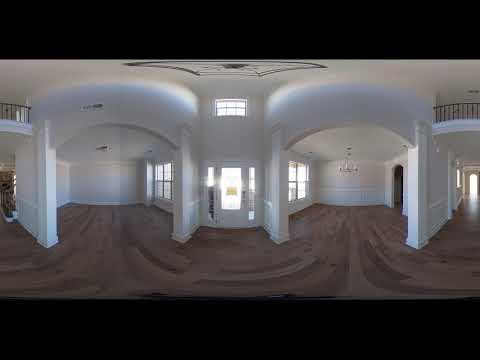The image depicts the grand interior of a luxurious, recently built mansion. The focal point is a great room with soaring white walls and ceilings that give the impression of a cathedral. Upon entering the home, you are greeted by an expansive, almost monstrous main living space. A striking black wire chandelier hangs centrally from the ceiling, illuminating the room.

The floor is an elegant mix of carpet and sweeping brown hardwood, adding a rich contrast to the predominantly white decor. Light floods in through a central doorway flanked by two narrow panels of glass, casting a soft glow throughout the space. The layout is symmetrical, featuring arched hallways and numerous walkways, doors, and windows that contribute to the open, airy atmosphere.

On either side of the main entrance are empty but inviting rooms. The left room has a frame window opening to the right, while the right room features a similar window opening to the left along with a ceiling-mounted candelabra and a narrow arched doorway possibly leading to a closet. Extending further, hallways on both sides lead to additional spaces, while above, a second-floor veranda with black railings overlooks the great room.

This grand, vacant home, exuding a unique and fresh aesthetic, is marked by its cavernous spaces, symmetry, and blend of modern and classical architectural elements.